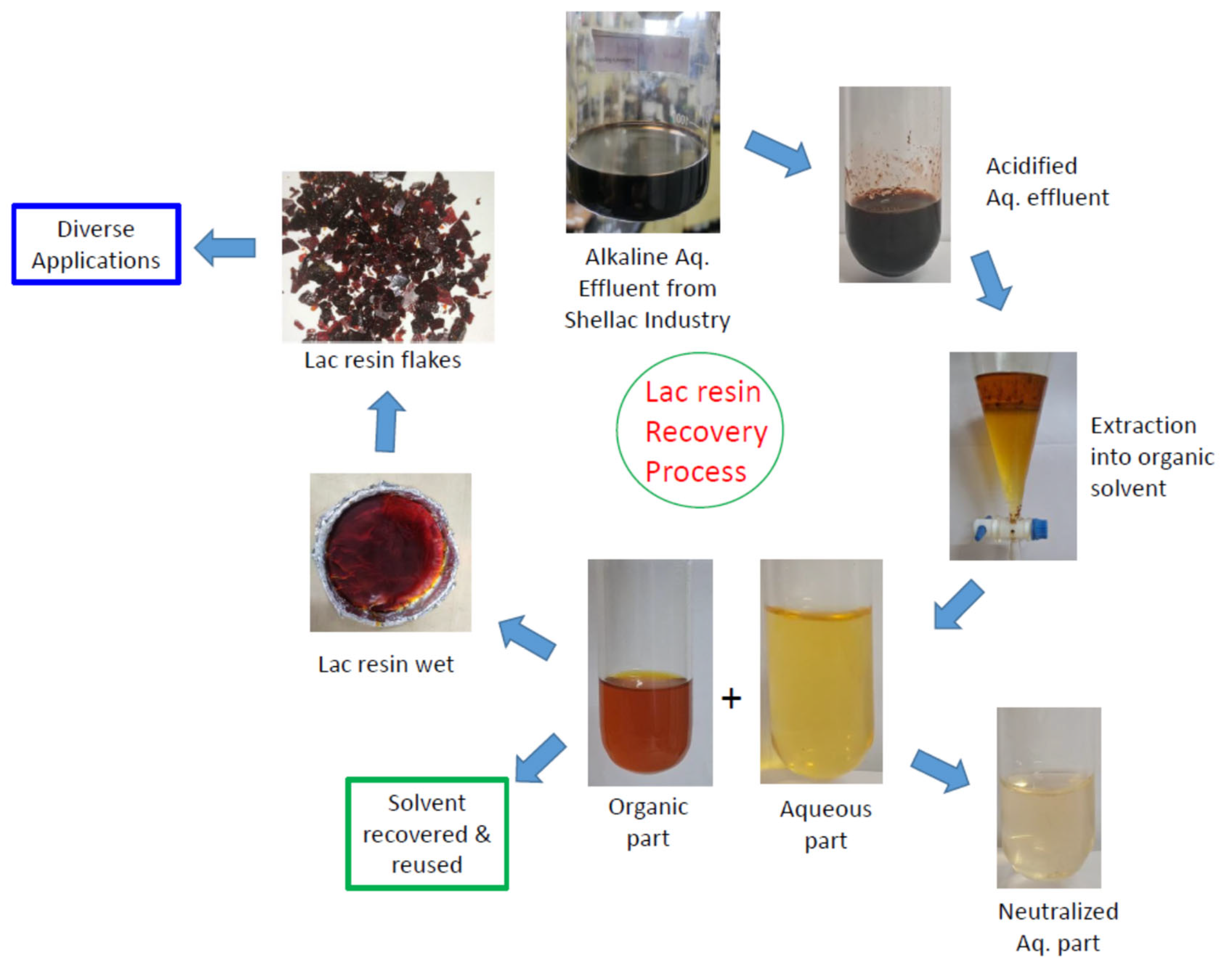This image is a detailed flowchart titled "Lack Resin Recovery Process," prominently labeled in a green circle with red text at the center. Starting from the top and moving clockwise, it features eight smaller photos each depicting different stages of the process. The first image shows a beaker filled with black fluid. Next is a test tube containing the same black fluid, followed by a separatory funnel with an amber top layer and a yellowish bottom layer. Continuing clockwise, there are two images centered at the bottom: one with a separated darker liquid and the other with a separated lighter liquid. The sequence proceeds to a small pie dish containing amber oil and then to dark resin flakes. The final image, branching off to the bottom right, displays a clearer liquid in a test tube. Blue arrows guide the flow between these images.

Each stage is annotated with descriptive text such as "Lack Resin Wet," "Lack Resin Flakes," "Diverse Applications," "Alkaline Ac Affluent from Shellac Industry," "Aquified Ac Affluent," "Extraction into Organic Solvent," "Neutralized Ac Part," "Aqueous Part," and "Organic Part." Additional text boxes highlight parts of the process, mentioning that the solvent is recovered and reused, and noting various applications. The entire chart is set against a white background, making the detailed steps of the lack resin recovery process clear and comprehensible.